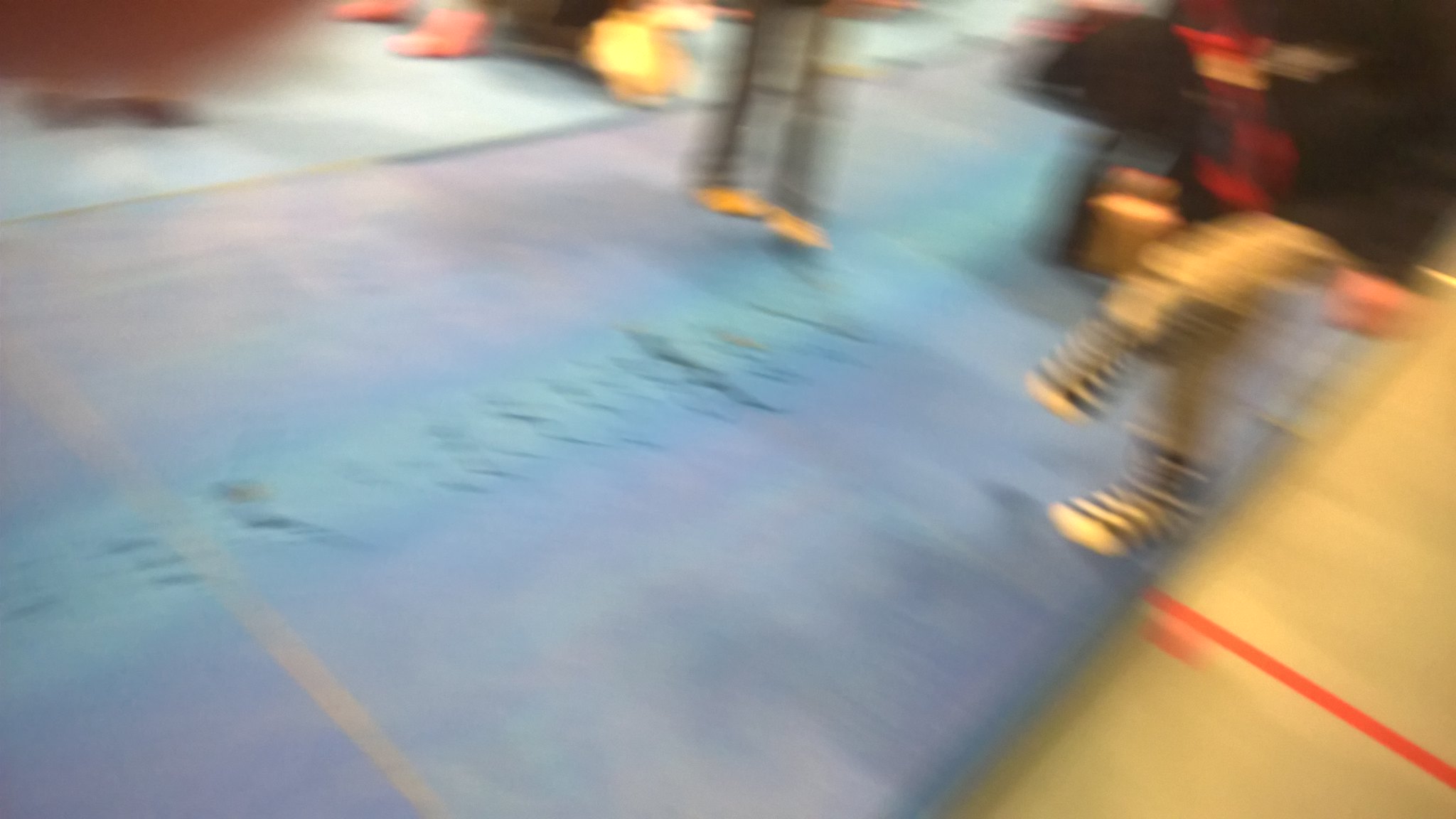In this very blurry image, the scene depicts a floor or mat area, possibly inside a store or on a sidewalk, dominated by a long blue rug or mat with varying shades of blue. There's a distinctive red line in the middle of the floor. The image features multiple people, albeit unclear due to the blurriness, which might include the photographer's thumb partially covering the camera in the top left corner, the only relatively clear element. In the center and upper parts of the image, two individuals appear to be dancing or standing: one wearing a red shirt with blue and white striped socks and another in yellow socks. There are also mentions of what could be yellow pants with possibly black striped socks. The floor's design transitions from blue in the central and left areas to a more lit-up yellow section on the right. Additional colorful elements, like someone purportedly with pink boots, are also vaguely visible in the blurry background. The overall scene suggests movement as the camera appears to have been in motion while the picture was taken.